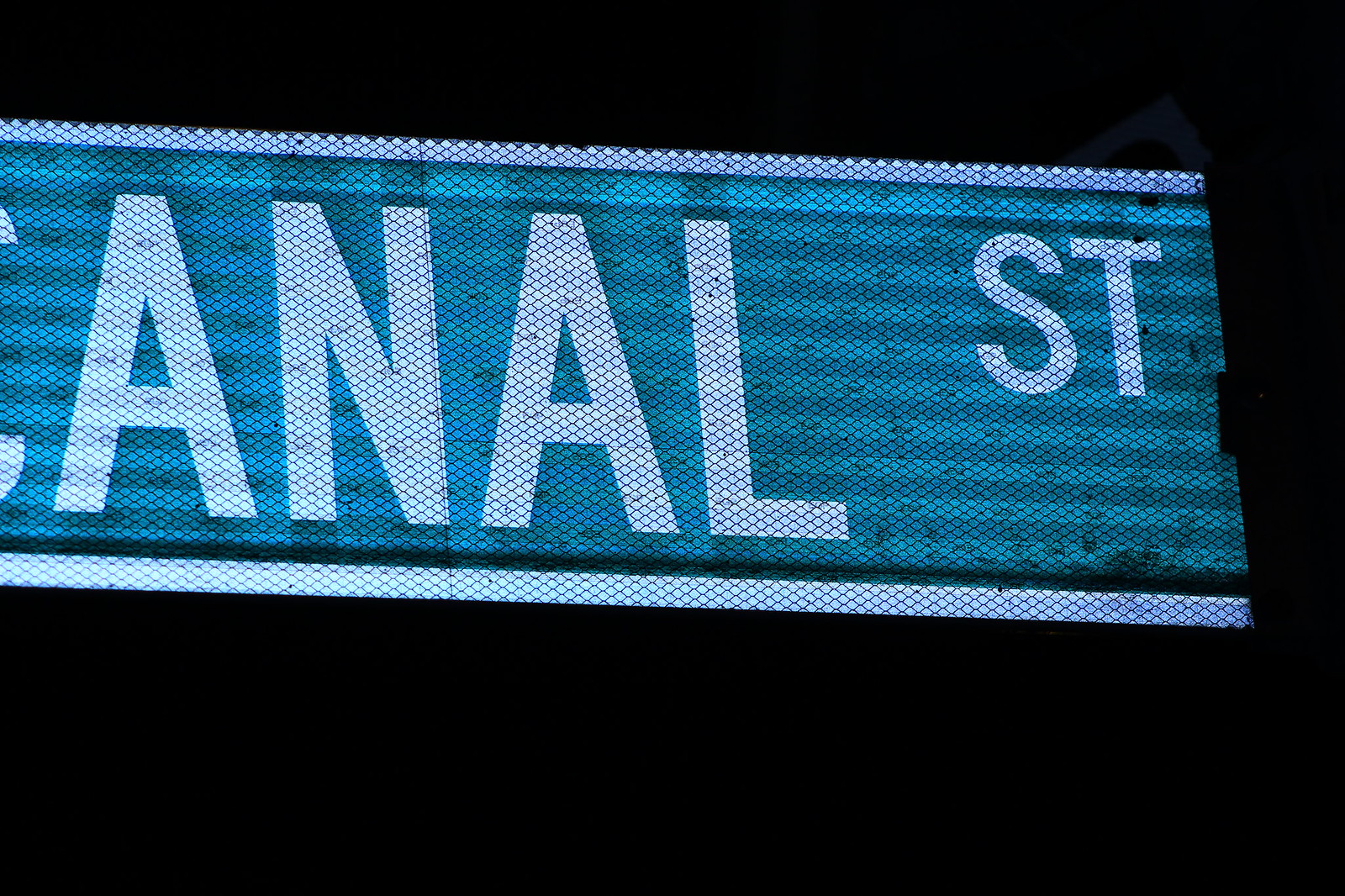The image features a digital sign with the text "Canal Street." The sign's design showcases a well-organized arrangement of colors and shapes. The topmost bar of the sign is white, followed by a light blue bar beneath it that transitions into a pattern of darker blue squares. The bottom section of the sign is entirely white. In the middle of this section, the word "Canal" is prominently displayed in bold letters. To the top right, the abbreviation "St." for "Street" is featured. Additionally, there are some darker, black markings concentrated at the bottom right corner of the sign, appearing as cross-marks or hatches. A distinct black line runs horizontally across the sign, further emphasizing the division of colors and sections. The overall appearance includes sporadic darker spots, adding subtle texture to the sign.